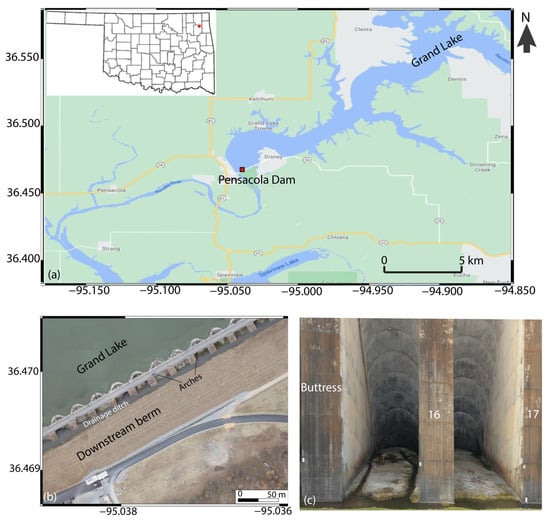The image is a composite of three distinct sections. The top section features a detailed map highlighting the Pensacola Dam and Grand Lake. The map is marked with coordinates on the left (ranging from 36.550 to 36.400) and along the bottom (from -95.150 to -94.850), providing precise geographical context. Additionally, a black line drawing with similar coordinates is superimposed on the upper left corner, further detailing the area. 

Below this, the lower left section (labeled B) presents an aerial view of Grand Lake, showcasing the downstream berm with visible arches and a road surrounded by green and brown terrain. This section also includes coordinates along the left side (36.469 at the top to 36.40 at the bottom) and at the bottom (95.038 on the left to 95.036 on the right). 

In the lower right section (labeled C), there is an image resembling a tunnel or canal with structural details marked by "buttress" and numbered beams labeled 16 and 17, indicating part of the dam's infrastructure.

Overall, this comprehensive triptych image provides a detailed geographical and structural overview of the Pensacola Dam and its surroundings, featuring both a map and photographic representations.